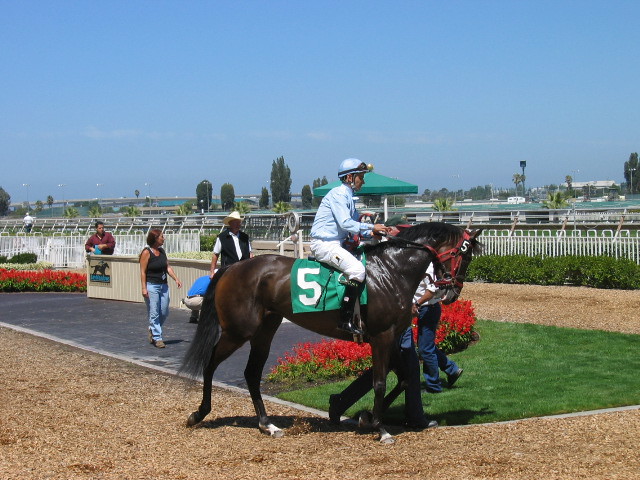In this vibrant photograph taken outdoors, perhaps at a prestigious horse derby such as the Kentucky Derby, the focal point is a striking, shiny, dark brown horse with a black mane and tail. This magnificent creature exudes vitality and strength, evidenced by its well-oiled, muscular frame. The horse is adorned with a red head guard and is draped in a green saddlecloth displaying the number five in bold white.

Astride the horse is a jockey, attired in a light blue helmet topped with goggles, a matching long-sleeve shirt, white pants, and knee-high black boots. His foot is secured in the stirrup as he looks downward, possibly contemplative or simply focused on his mount.

Adjacent to the horse, a person in black pants and a glimpse of a blue shirt walks alongside the animal. Encircling this scene is a straw-covered walkway bordered by lush green grass and vibrant red flowers, with a central stand prompting activity and interest. 

In the background, diverse characters populate the scene: a woman in blue jeans and a black tank top, a man bent over wearing beige pants and a blue shirt, another man sporting a black vest over a white shirt topped with a beige cowboy hat, and another individual in a burgundy shirt standing by a large beige bin featuring a horse graphic.

Further out, white fencing, additional seating areas, bushes, and a plethora of red flowers blending into the scene, while the horizon showcases trees and small buildings beneath a clear blue sky. This meticulously captured moment radiates the energy and anticipation typical of a racetrack setting.